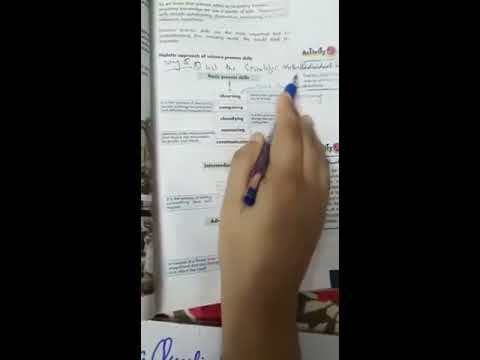This image is a wide rectangular photograph featuring a central, slightly blurry snapshot of a right hand with light brown skin holding a blue pen. The hand emerges from the bottom right, positioned palm down with the thumb on the left and the pinky finger towards the top. It is resting atop a white piece of paper, which seems to be part of a children's homework book, filled with small, black, unreadable text, possibly word problems. The surrounding area of the image to the left and right is entirely black, contrasting sharply with the white page and the brown skin tone. Beneath the hand, part of the patterned surface, with green, white, and red colors, on which the book rests, is visible. The overall scene suggests an educational context, possibly a screenshot from a video tutorial.